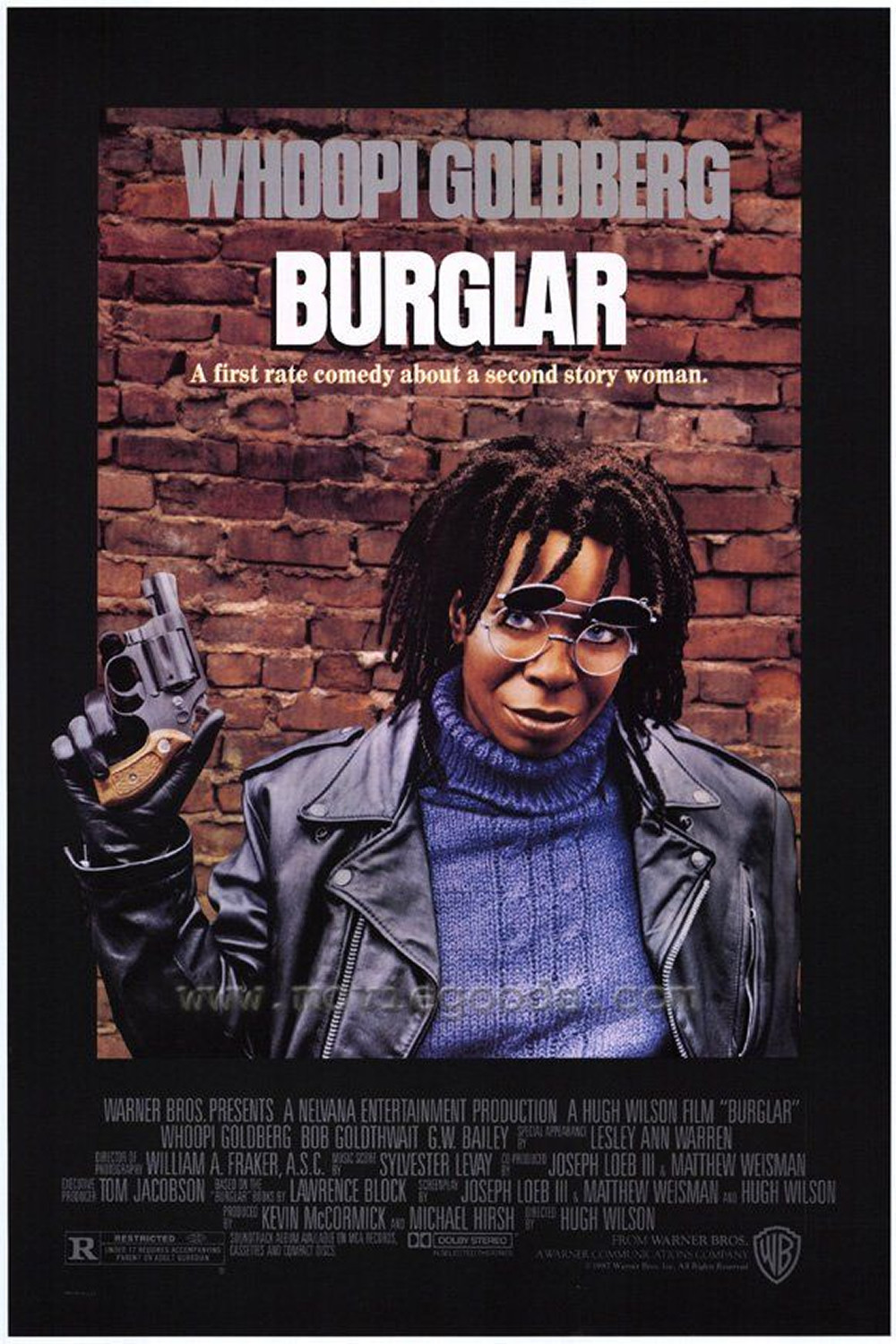The image is a full-color, computer-animated movie poster featuring a younger Whoopi Goldberg. The portrait-format poster is for the movie **Burglar**, prominently titled at the top with the tagline, "A first-rate comedy about a second-story woman." Whoopi Goldberg is shown from her midsection upward. She dons a black leather motorcycle jacket over a blue turtleneck sweater. Her hair is styled in short dreads, and she wears distinctive glasses with the lenses flipped up, revealing light-colored frames. In her right hand, she holds a leather glove and a small revolver with a rotary center barrel and a wooden handle. The backdrop hints at a red brick building. Toward the bottom, credits include mentions of Warner Brothers and Nelvana Entertainment Production, along with various other names. The movie is rated R, and there is a barely legible website watermark across her jacket.